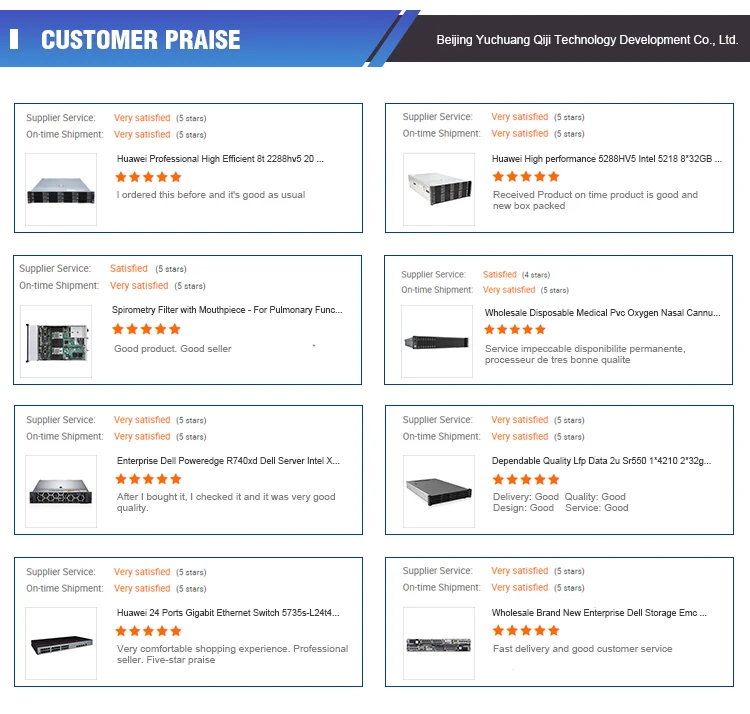The web page features a clean white background, providing a minimalist and modern look. At the top of the page, a vibrant blue rectangular box with a creatively jagged, diagonally cut end stands out. This blue box partially overlaps a smaller black rectangular box underneath. Bold white text on the blue box reads "Customer Praise," while the black box below displays "Beijing Yucheng Qiji Technology Development Co Ltd" in white text.

The body of the page is organized into two rows, each containing four sections, making a total of eight rectangular sections outlined in dark blue. Each section showcases a product and its reviews in a structured layout.

**First Row:**
1. **Huawei Professional High-Efficient 8T2288HV520**
   - Supplier Service: Very Satisfied, 5 stars
   - On-Time Shipment: Very Satisfied, 5 stars
   - Review: "I ordered this before, and it's good as usual."
   - Rating: ⭐⭐⭐⭐⭐

2. **Spirometry Filter with Mouthpiece for Pulmonary Function**
   - Supplier Service: Satisfied, 5 stars
   - On-Time Shipment: Very Satisfied, 5 stars
   - Review: "Good Product, Good Seller."
   - Rating: ⭐⭐⭐⭐⭐

3. **Enterprise Dell PowerEdge R740XD Dell Server Intel X**
   - Supplier Service: Very Satisfied, 5 stars
   - On-Time Shipment: Very Satisfied, 5 stars
   - Review: "After I bought it, I checked it, and it was very good quality."
   - Rating: ⭐⭐⭐⭐⭐

4. **HealAway 24 Ports Gigabit Ethernet Switch 5735S-L24T4**
   - Supplier Service: Very Satisfied, 5 stars
   - On-Time Shipment: Very Satisfied, 5 stars
   - Review: "Very Comfortable Shopping Experience Professional Seller, 5 star praise."
   - Rating: ⭐⭐⭐⭐⭐

**Second Row:**
1. **HealAway High Performance 5288HV5 Intel 52188 Star 32GB**
   - Supplier Service: Very Satisfied, 5 stars
   - On-Time Shipment: Very Satisfied, 5 stars
   - Review: "Received Product on Time, Product is Good, and New Box Packed."
   - Rating: ⭐⭐⭐⭐⭐

2. **Wholesale Disposable Medical PVC Oxygen Nasal Cannula New**
   - Supplier Service: Satisfied, 4 stars
   - On-Time Shipment: Very Satisfied, 5 stars
   - Review: "Service Impeccable, Disponibilit Permanente Processor de Trebon Qualite."
   - Rating: ⭐⭐⭐⭐⭐

3. **Dependable Quality LFP Data T2USR550**
   - Supplier Service: Very Satisfied, 5 stars
   - On-Time Shipment: Very Satisfied, 5 stars
   - Review: "Delivery Good, Quality Good, Design Good, Service Good."
   - Rating: ⭐⭐⭐⭐⭐

4. **Wholesale Brand New Enterprise Dell Storage EMC**
   - Supplier Service: Very Satisfied, 5 stars
   - On-Time Shipment: Very Satisfied, 5 stars
   - Review: "Fast Delivery and Good Customer Service."
   - Rating: ⭐⭐⭐⭐⭐

This detailed layout effectively highlights user reviews and product ratings, providing potential customers with insightful feedback.